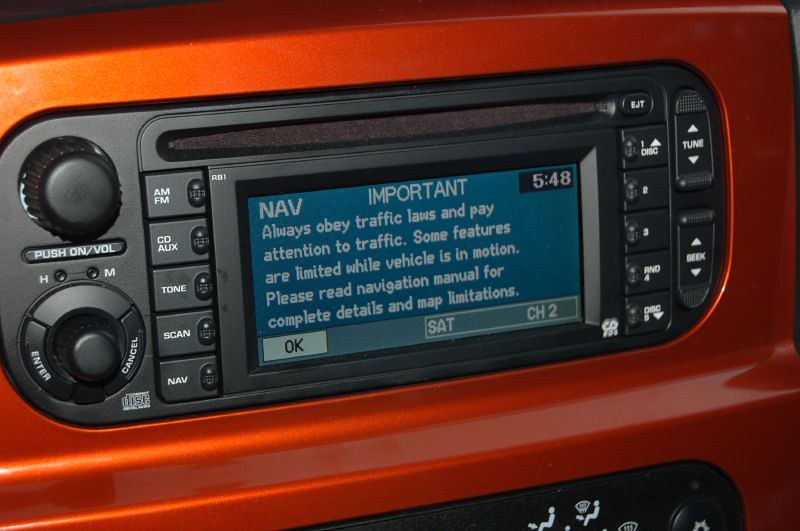This detailed photograph captures the entertainment console on the dashboard of a modern automobile, predominantly showcasing its car radio system. The background color of the car is likely orange, aligning with the hints of orange seen around the console. The radio unit itself is black and features a compact yet comprehensive array of controls.

On the left side of the console, there are multiple knobs designed to control power, volume, and other functionalities. Specific buttons are assigned to various functions such as AM/FM, CD/Auxiliary, Tune, Scan, and Navigation. Below these knobs is a toggle switch used for Enter and Cancel operations.

Centrally located on the console is a blue navigation screen that displays a critical safety message in white text: "Important. Always obey traffic laws and pay attention to traffic. Some features are limited while the vehicle is in motion. Always read the navigation manual for complete details and map limitations." Directly below this message is an OK button in a white box, and to its right, in a gray box, is an indicator reading "Sat CH2," signifying the satellite channel is set to channel 2. Additionally, the time "5:48" is visible in a black box set against the pale blue background of the screen.

On the far right of the console are further control buttons for tuning and seeking stations. The top row includes standard presets, with one labeled button featuring an arrow possibly for disk ejection. Another toggle button, "Seek," helps in finding stations, and these buttons show directional arrows for navigation through options.

Overall, this car radio is integrated into an entertainment system that includes radio, CD player, and navigation, exemplified by its detailed and user-friendly interface.